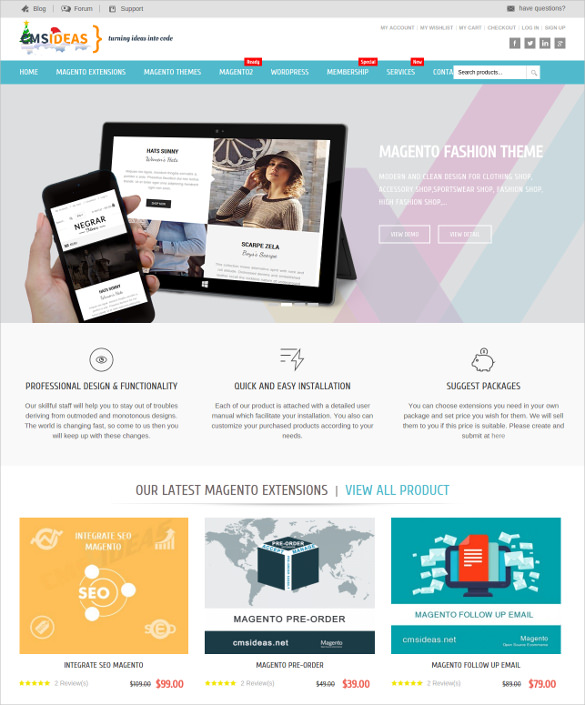This image, sourced from a website promoting EMS ideas and the transformation of concepts into code, depicts a multifaceted scene. At the forefront, a woman, identifiable by her pink-painted fingernails, holds a cell phone in her hand. The focal area also includes a picture frame showcasing another woman who appears to be around 32 years old, sporting a hat and dirty blonde hair.

Adjacent to the framed photo, there is text highlighting features of a "Magento Fashion Theme," which emphasizes professional design and functionality, as well as quick and easy installation. The description encourages users to suggest packages, allowing them to choose the necessary extensions and set their desired prices. Additionally, a "Magento Pre-Order" tab is visible, along with a promotional note for "Magento Follow-Up Email" priced at $79. The overall scene conveys a blend of technology, e-commerce, and personalized design options.